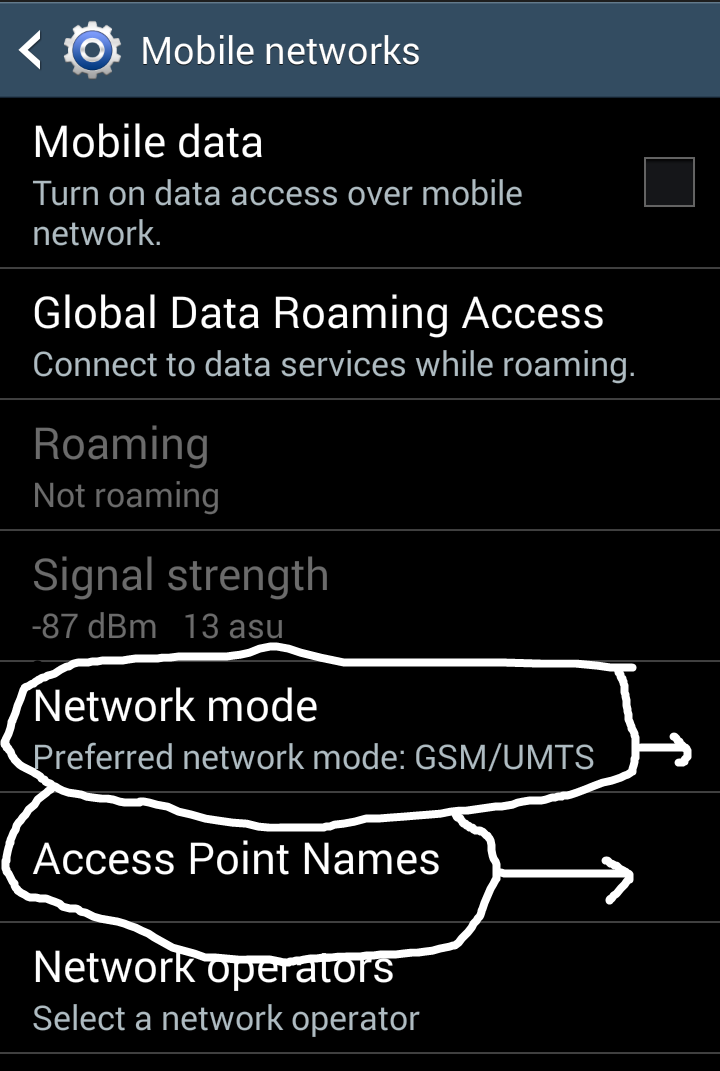This screenshot, captured in portrait mode, shows a mobile device's settings menu under "Mobile Networks." The content features a blue-gray header displaying "Mobile Networks," and the background transitions to black beneath this header. Several options are listed, each accompanied by relevant status indicators or checkbox options:

1. **Mobile Data:** An option to turn on data access over the mobile network, currently unchecked.
2. **Global Data Roaming Access:** An option to connect to data services while roaming.
3. **Roaming Status:** Displays "Not Roaming" in gray text, which is harder to read.
4. **Signal Strength:** Indicates "-87 dBm 13 ASU" in gray, making it somewhat challenging to discern.

The person who created the screenshot has highlighted specific entries with white handwritten markings and arrows:

- **Preferred Network Mode:** This entry is encircled with an off-center white oval and has an arrow pointing to the right, suggesting the need to click on it. The text reads "Preferred network mode: GSM/UMTS."
- **Access Point Names (APNs):** Similarly circled and marked with an arrow, indicating another clickable option.

Finally, under these highlighted entries is:

- **Network Operators:** An option to select a network operator.

Overall, the creator of this screenshot seems to have drawn attention to specific settings for adjusting the network mode and access point names under the "Mobile Networks" menu.